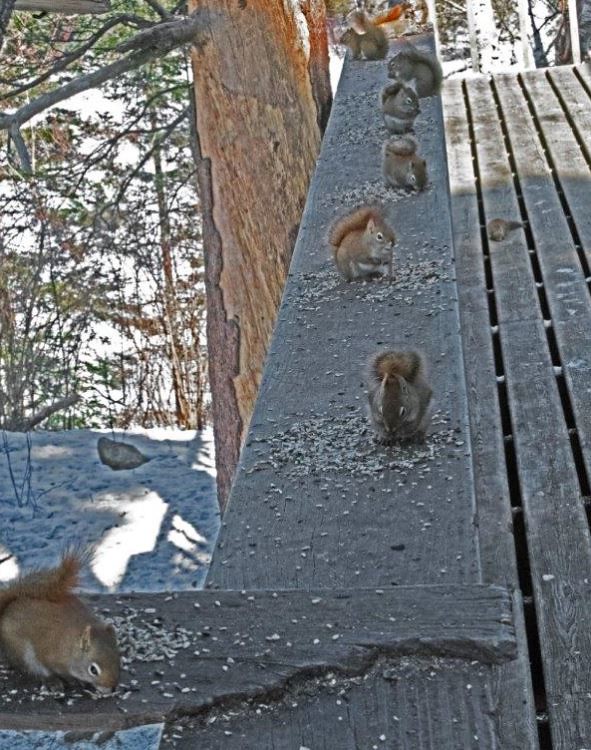The photo captures a weathered, unstained wooden deck situated outdoors, overlooking a snowy ground area. This deck seems to be set high, possibly a porch or railing, surrounded by trees with green leaves and brown bark. Despite the low-quality, somewhat fuzzy image, you can see a total of at least seven, possibly more, fluffy and well-fed squirrels, each varying in shades of brown and gray with distinctive fluffy tails and black eyes. The squirrels are scattered across the deck planks, enjoying piles of sunflower seeds or similarly shaped nuts. Each squirrel faces in differing directions, some look left, others right, and a few are directly facing the camera, creating a lively and dynamic scene.